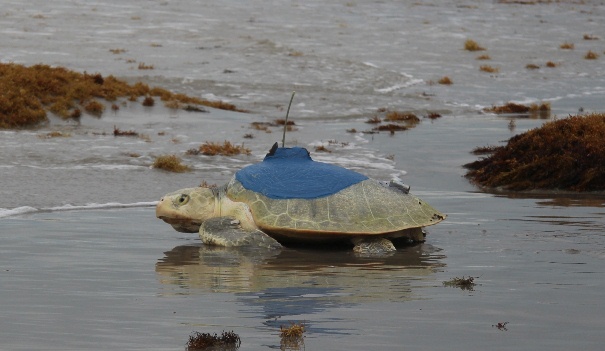In this outdoor photograph, a large tortoise is walking along a sandy, wet shore, partially wading through very shallow, gray water. The tortoise, which has a light green shell and darker green legs, is heading towards the left side of the image with its eyes open. A notable feature on the tortoise is a blue tagging device attached to the top of its shell; this device has a small antenna protruding from its center. Surrounding the tortoise, there are patches of brown, waterlogged vegetation, and small waves gently lap against the shore. In the background, further out to sea, the water becomes more turbulent, while areas of seagrass and brown grasses grow on small hills to the right and left. No people or text are visible in this serene, natural scene.